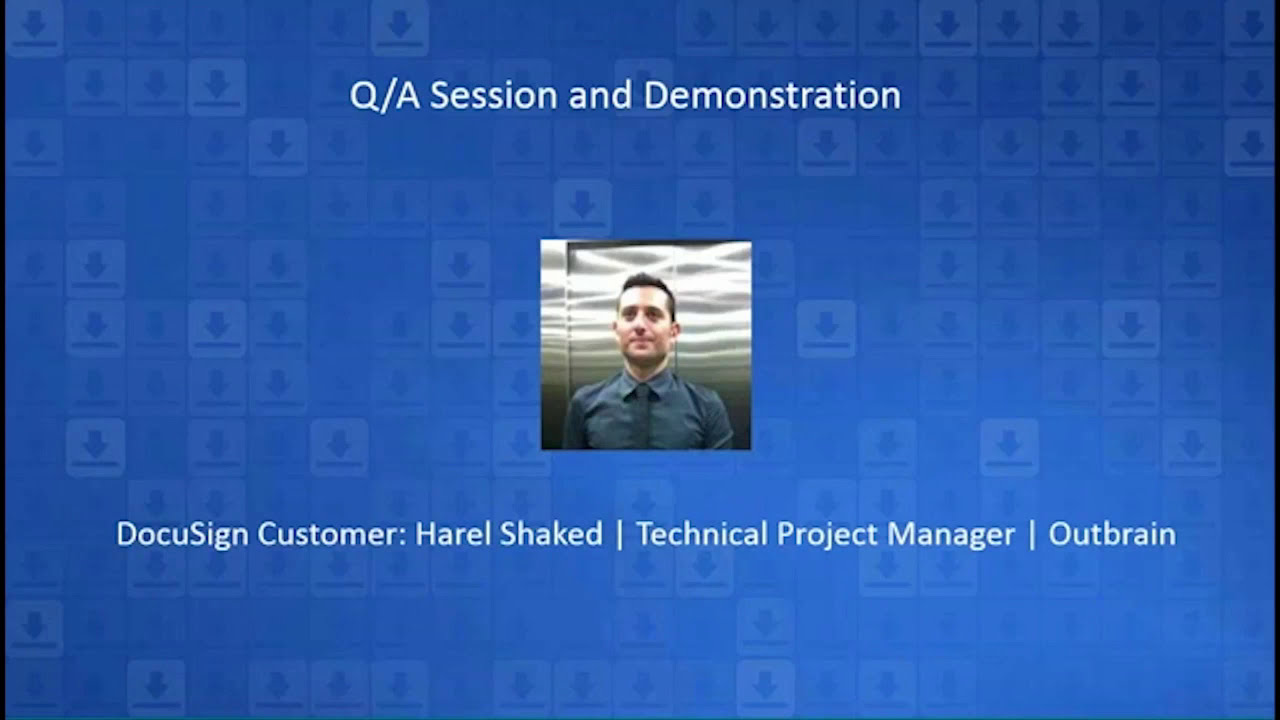This image is a screenshot of a presentation slide with a detailed blue patterned background composed of alternating translucent square tiles, each featuring a dark arrow pointing downward above a horizontal line. The top of the image displays the text "Q/A session and demonstration" in white font. Centrally positioned is a small square color photograph of a young, clean-shaven man with short hair. He is dressed in a grayish-blue collared shirt and a blue tie, and he stands in front of what appears to be a silver elevator, reflecting ceiling lights. Beneath the photograph, in white font, it reads: "DocuSign customer Harold Shaked, Technical Project Manager, Outbrain." The image includes shades of blue, white, black, silver, tan, and a hint of gray.